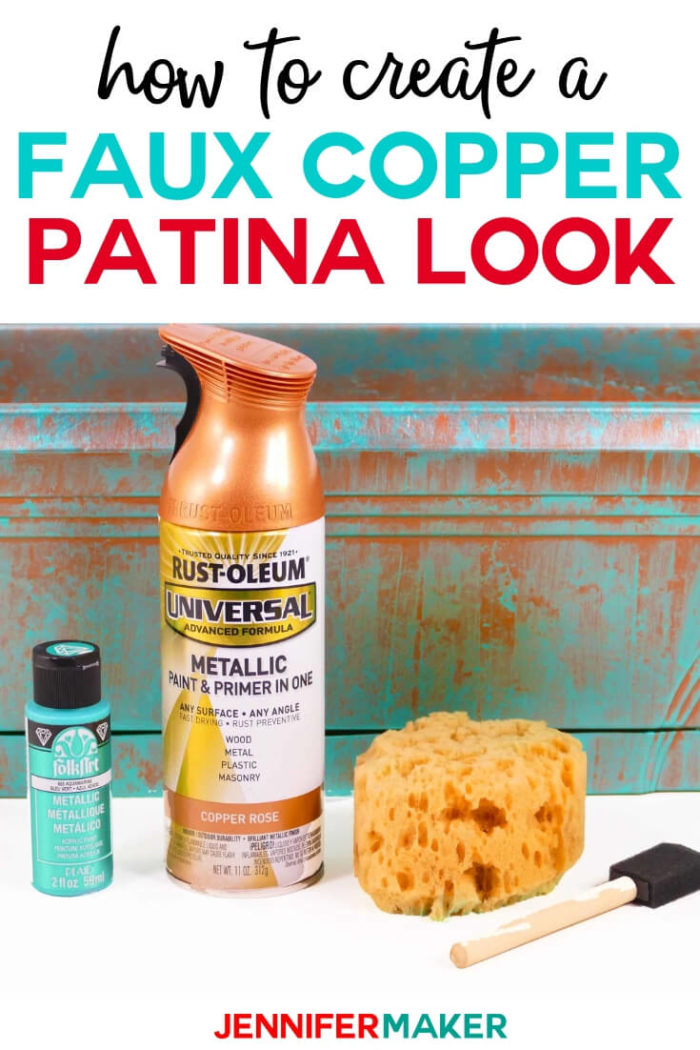This advertisement features a detailed, step-by-step guide on how to create a faux copper patina look. The instructional poster heading combines black, blue, and red text that reads "How to create a faux copper patina look." At the center of the image, there are several essential tools displayed on a white surface. These include a copper-colored can of Rust-Oleum Universal Advanced Formula Metallic Paint and Primer in One, which features an orange label with golden accents and the word "Universal" prominently highlighted. Next to the Rust-Oleum can is a bluish-green bottle with a black cap labeled as a metallic product, though the exact name is not entirely legible.

Adjacent to these items, there is a sponge and a small foam brush with a wooden handle and a black tip, indicating the tools necessary for applying the patina effect. The bottom of the poster prominently displays the name Jennifer Maker, with "Jennifer" in red and "Maker" in green, emphasizing the source of this how-to guide.

In the background, a surface showcasing the desired faux copper patina look is visible, characterized by a blend of greenish, metallic hues interspersed with reddish-orange streaks, reminiscent of aged copper. The overall design of the advertisement merges instructional content with a visual reference to the finished effect, ensuring clarity for those attempting to recreate the look.